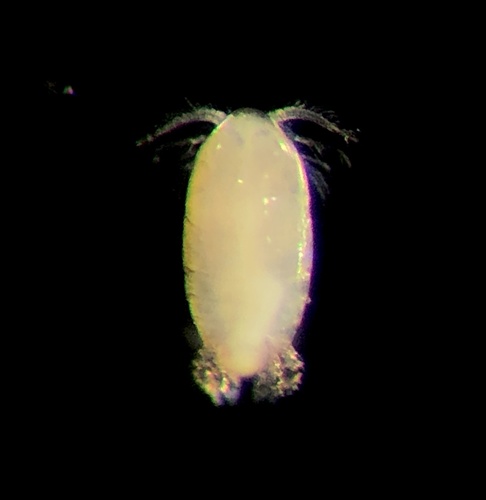The image depicts an extreme close-up of a small insect-like organism positioned vertically against a solid black background, likely taken under a microscope. The main body of the insect is an oval-shaped, pale yellow, and slightly translucent, with a shiny appearance. Prominent features include two curved, beige-colored antennae extending from the top, adorned with fine, almost prickly hairs. These antennae arch downward slightly. Subtle creases along the sides of the body suggest segmentation. At the bottom of the bug, there are two indistinct clumps that appear fuzzy and may have tiny fibers, but they do not resemble clear, solid legs or limbs. Additionally, there's a small, translucent dot with a red and green hue diagonally positioned to the object's upper left, perhaps another microscopic subject.